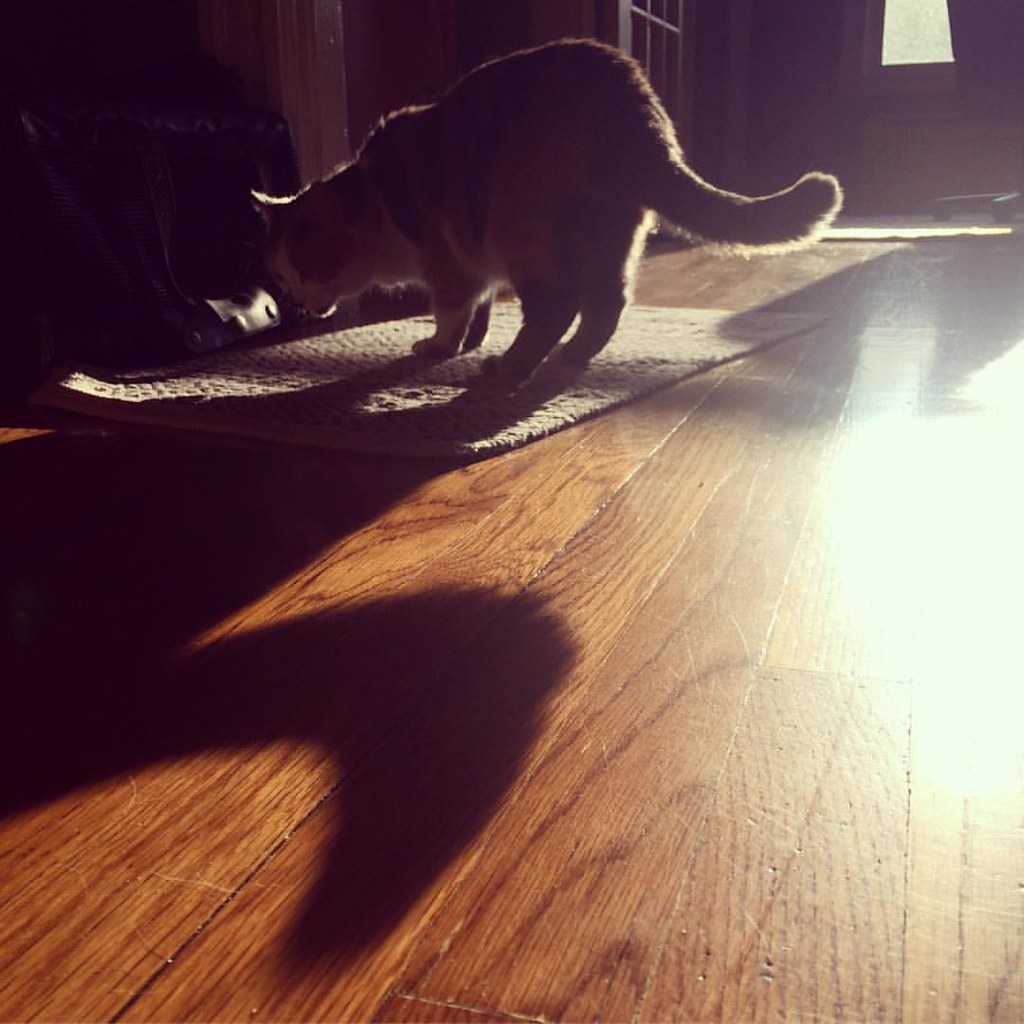The photograph captures a cat in a dimly lit room, with the primary light source being sunlight streaming through a window in the upper right-hand corner. The bottom half of the window is visible in the far distance, and the sunlight illuminates the golden brown hardwood floor, casting a stark shadow. The cat, positioned in the upper third of the image, is on all fours with its back hunched and its head bent downwards, seemingly focused on something shiny on the light beige wool rug beneath it. Its tail is curved upwards, creating an elongated and distinct shadow stretching towards the lower left-hand side of the photo. The cat's brownish or tawny fur stands out against the shaded backdrop. The viewer’s perspective is level with the cat, capturing the scene closely as if lying on the floor. The detail of the wooden floor, with its visible grains, adds to the overall texture and depth of the image, and a brown wall is perceptible behind the cat, enhancing the composition.